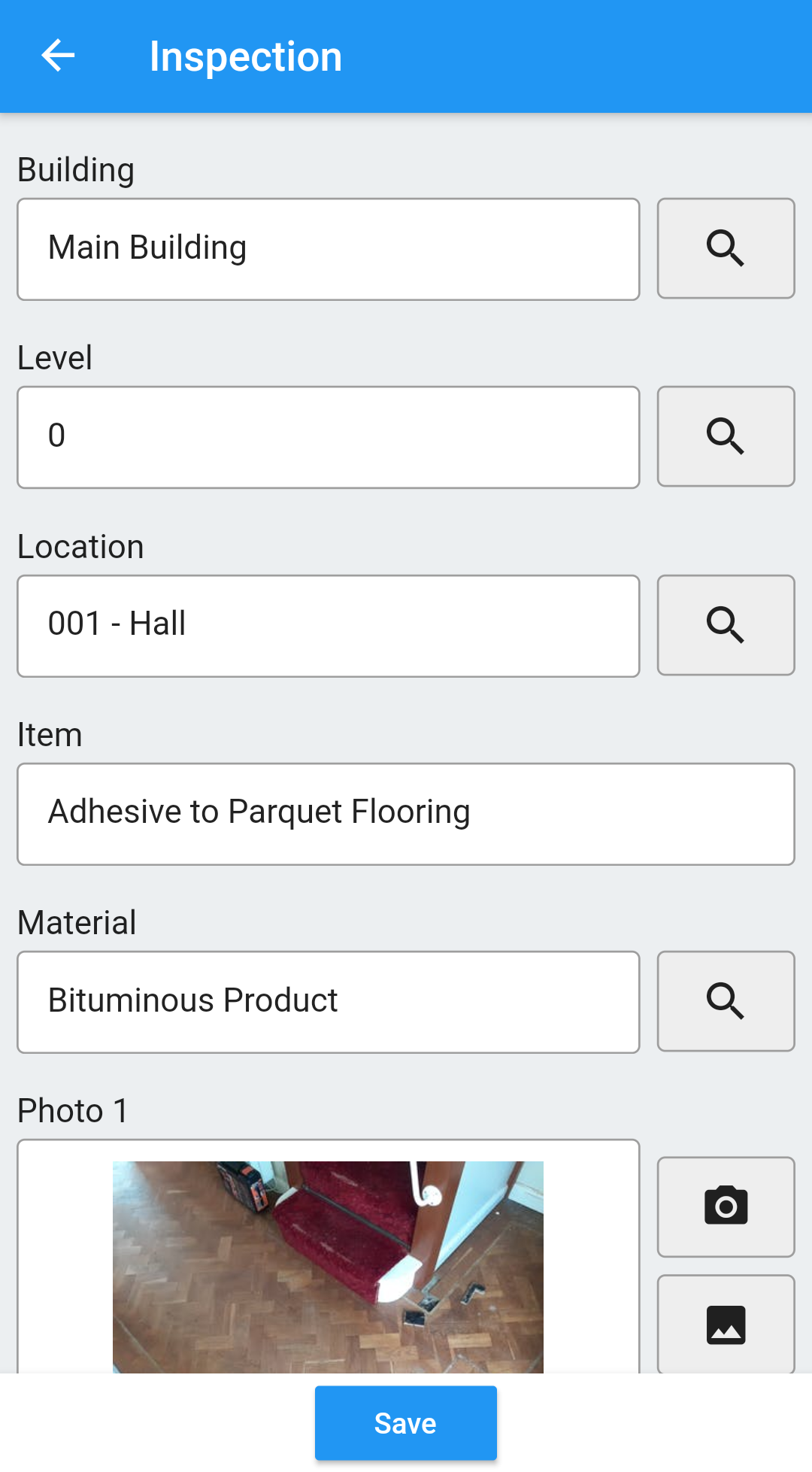This image is a cell phone screenshot of a record-keeping application displaying an inspection form. The interface features a light gray background, creating a clean and simple look. At the very top, a blue rectangular bar spans the width of the screen, with the word "Inspection" left-justified in white text. To the left of this title, a white left-pointing arrow icon indicates the option to return to a previous menu.

Immediately below this blue bar, the form begins on the light gray background. The first field is labeled "Building," with the entry "Main Building" filled in; there is a magnifying glass icon to the right of this entry, indicating a search function. The next field down is labeled "Level," containing the entry "0," also with a magnifying glass icon on the right.

The third field is "Location," filled with the entry "001-hall," and again includes a search icon to the right. Following this is the "Item" field, with "Adhesive to parquet flooring" entered. The fifth field is labeled "Material," showing "Bituminous product" as the entry, with a search icon positioned on the right as well.

Beneath these text fields, there is a section labeled "Photo 1" displaying an image of wooden parquet flooring. Adjacent to this image are two functional buttons: the top button features a camera icon, allowing the user to capture a new photo, while the lower button shows a photo icon for uploading an existing image.

At the bottom center of the screen, a prominent blue rectangle button with the word "Save" in white text is visible, providing the option to save the entered information.